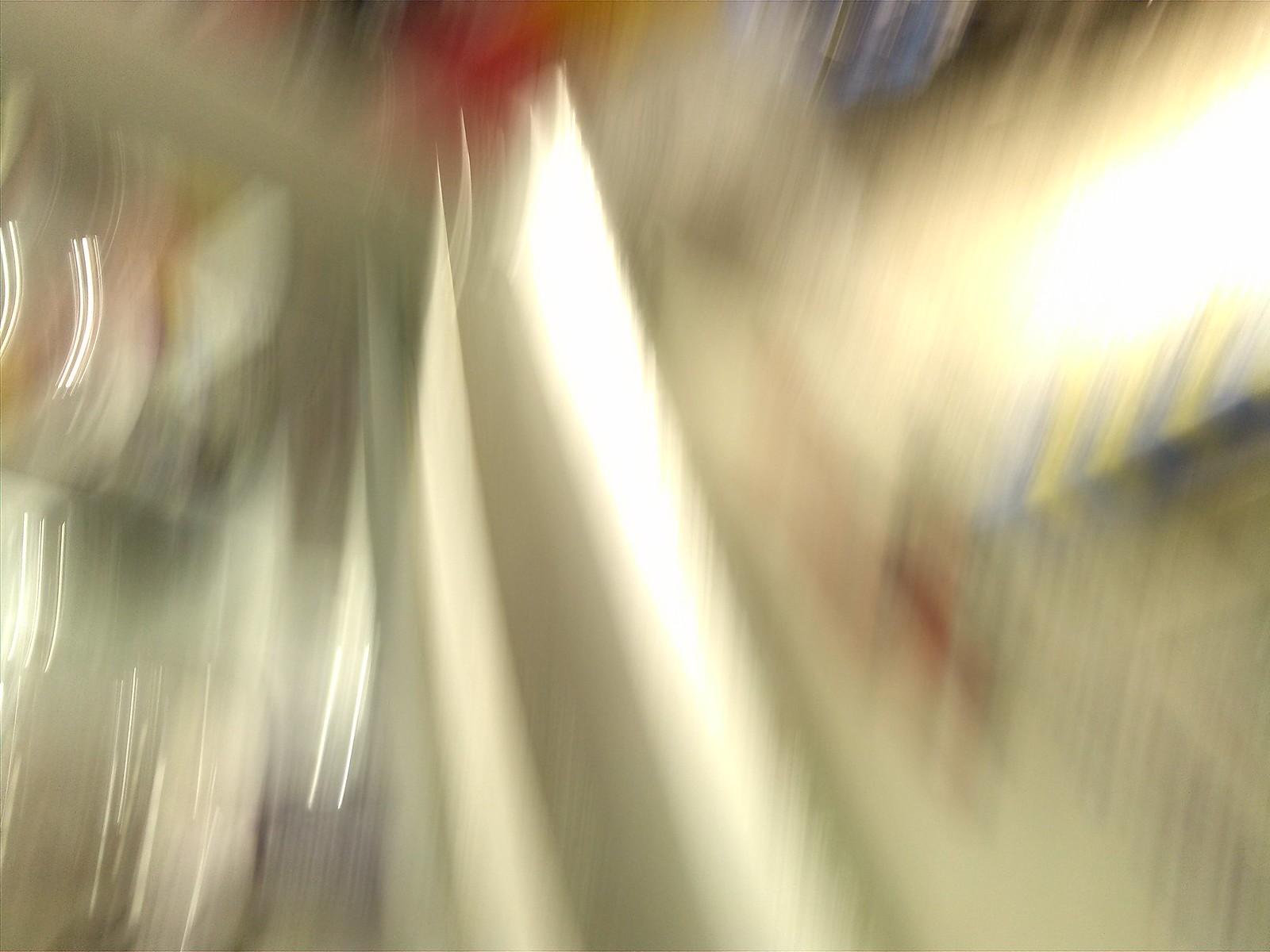This highly blurred photograph predominantly features a wash of white, suggesting a significant presence of light at the location where the photo was taken. The blurred lights are smeared across the image, creating streaks that give the impression of a brightly illuminated scene. Amidst the blurriness, there's a discernible horizontal rectangle marked with blue, yellow, and black stripes, though its precise nature remains indiscernible. Additional smudges of blue appear sporadically throughout the image, with notable patches at the top and on the left side. A hint of red is also visible towards the top, but the overall indistinct quality of the photo makes further details elusive.